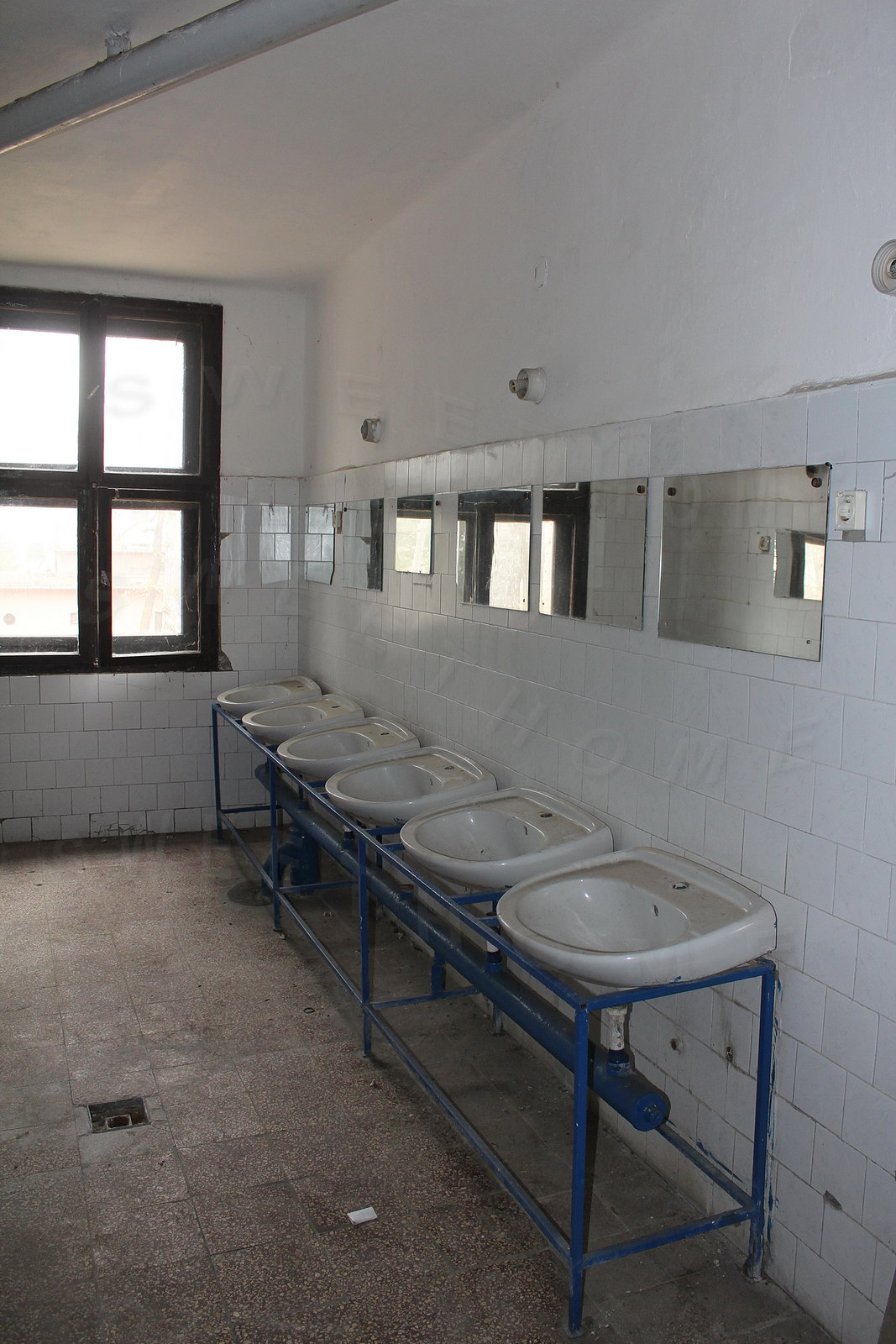The image depicts a rundown public restroom, potentially located in a local park or an old school. The floor features a gray, square brick tile pattern with a missing drain cover in the center. The walls are lined with white tiles, which appear rusty and dirty, particularly near the bottom where some tiles are grimy and chipped. The focal point of the restroom is a row of six U-shaped sinks, each mounted on a blue metal shelf with matching blue, black, and silver pipes underneath. However, these sinks are notably missing their faucet fixtures, rendering them non-functional. Above the sinks, plain mirrors are mounted on the wall. At the end of the room, there's a window divided into four sections by a dark brown or black frame. Overall, the space has a neglected and poorly maintained appearance, suggesting it is only checked on infrequently.